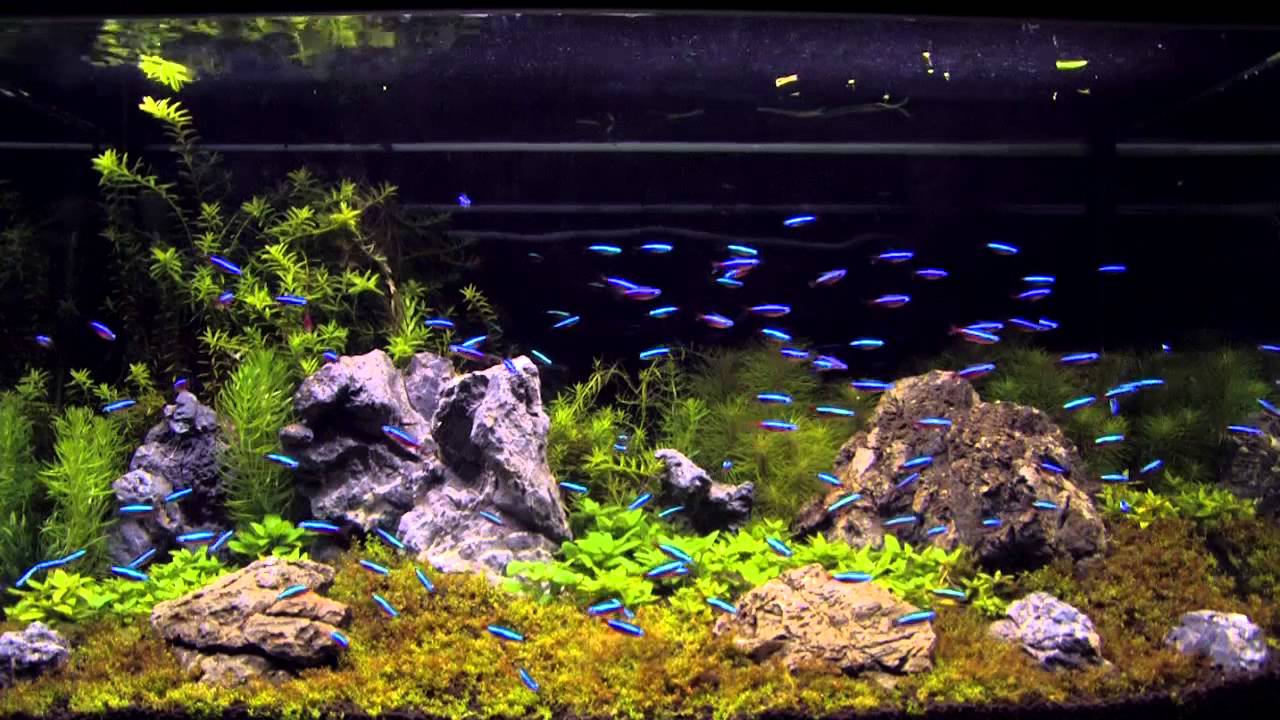The image depicts a large, rectangular aquarium with a black background. The bottom of the tank is decorated with a mixture of green and brown mossy plants, with the green hues being more prominent in the center and tapering to a brownish tint on the right. Numerous rocks of varying sizes and colors are scattered throughout the base, including a massive, craggy gray rock on the left and a significant brown rock on the right.

Emerging from the back of the aquarium are long plants that stretch upwards, mingling with smaller fronds of grass that extend towards the top of the tank. The middle of the image features taller vegetation and larger rocks, adding a dynamic vertical element to the scene.

A school of small, thin fish with fluorescent blue tops and reddish bellies swims together in a group, primarily staying below the midline of the tank. The array of details within the aquarium, from the lively fish to the diverse plant life and varying rock formations, creates an intricate and vibrant underwater tableau.